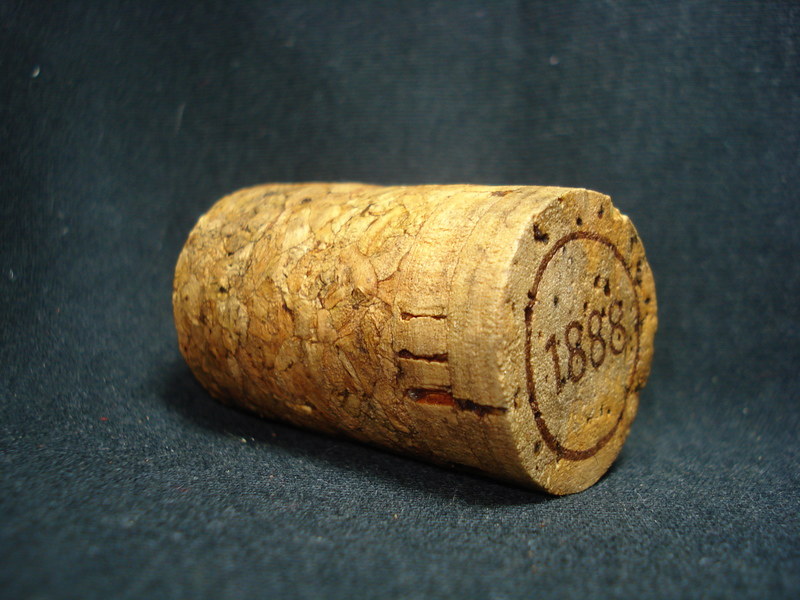This is an extreme close-up photograph of a wine cork placed on a textured, bluish-gray surface that resembles carpet. The background fabric has a lot of dimension, with different specks of gray and other tiny colors, creating a visually rich backdrop, though it is mostly blurred to emphasize the cork. The cork itself is cylindrical and made of traditional cork material, displaying a detailed texture that ranges from smooth on top to rougher towards the bottom. The top of the cork is particularly smooth, etched with a stamp that reads "1888," and features a few small divots. Just below the top, there are two slightly notched bands that are relatively smoother compared to the rest of the cork. Below these bands, the cork's texture becomes more pronounced with rough and uneven pieces. Some red slots and scratches can also be observed around it, enhancing the sense of age and use.